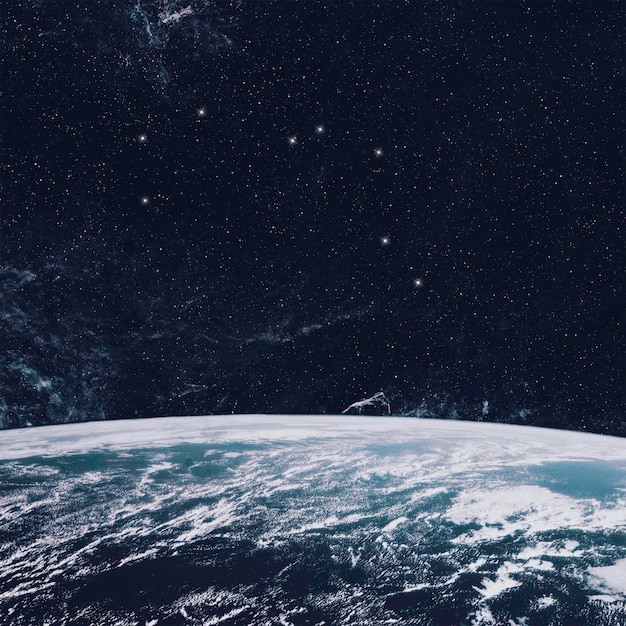This image appears to be a detailed, computer-generated view taken from space, capturing an Earth-like planet in low orbit. The lower half of the image features the planet which is predominantly blue, suggesting a vast ocean with no visible landmasses. The surface is covered in white, puffy clouds, enhancing the planet's vibrant, Earth-like appearance. Above the planet, the starry expanse of space unfolds, characterized by a deep, inky navy background scattered with numerous small, white stars. Among these stars, eight larger and brighter ones stand out, seemingly forming an almost M-shaped constellation, reminiscent of well-known star patterns such as the Big Dipper or Leo. Additionally, a hazy, smoky region in the distance might suggest galaxy formation or atmospheric phenomena. Overall, the image beautifully contrasts the serene, cloud-covered planet against the vast, star-filled emptiness of space.